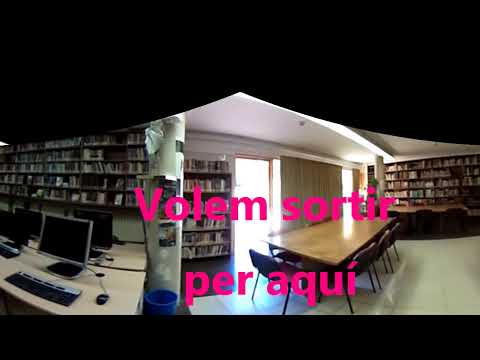This panoramic image captures a detailed view of a large library. The left side of the image features a long bookshelf brimming with books, opposite to which are two tables arranged parallelly, each hosting rows of computers with monitors, mouses, and keyboards facing back-to-back, allowing seating on either side. Next to these computer tables is a blue garbage can, placed near a support column. As the view shifts to the right, there is a large wooden table surrounded by chairs, illuminated by sunlight filtered through yellow curtains covering glass doors. Another wooden table and additional chairs are visible on the far right, set against another extensive bookshelf. The ceiling is painted white, with a strip of light running through its center, and the floors are a whitish hue. Over the image, in pink text, is a message in Spanish reading "Volem sortir per aquí," meaning "We want to exit here." The image is framed with a thick black border, which peaks at the top center, mimicking a mountain shape, while the bottom edge of the border remains parallel across the width.